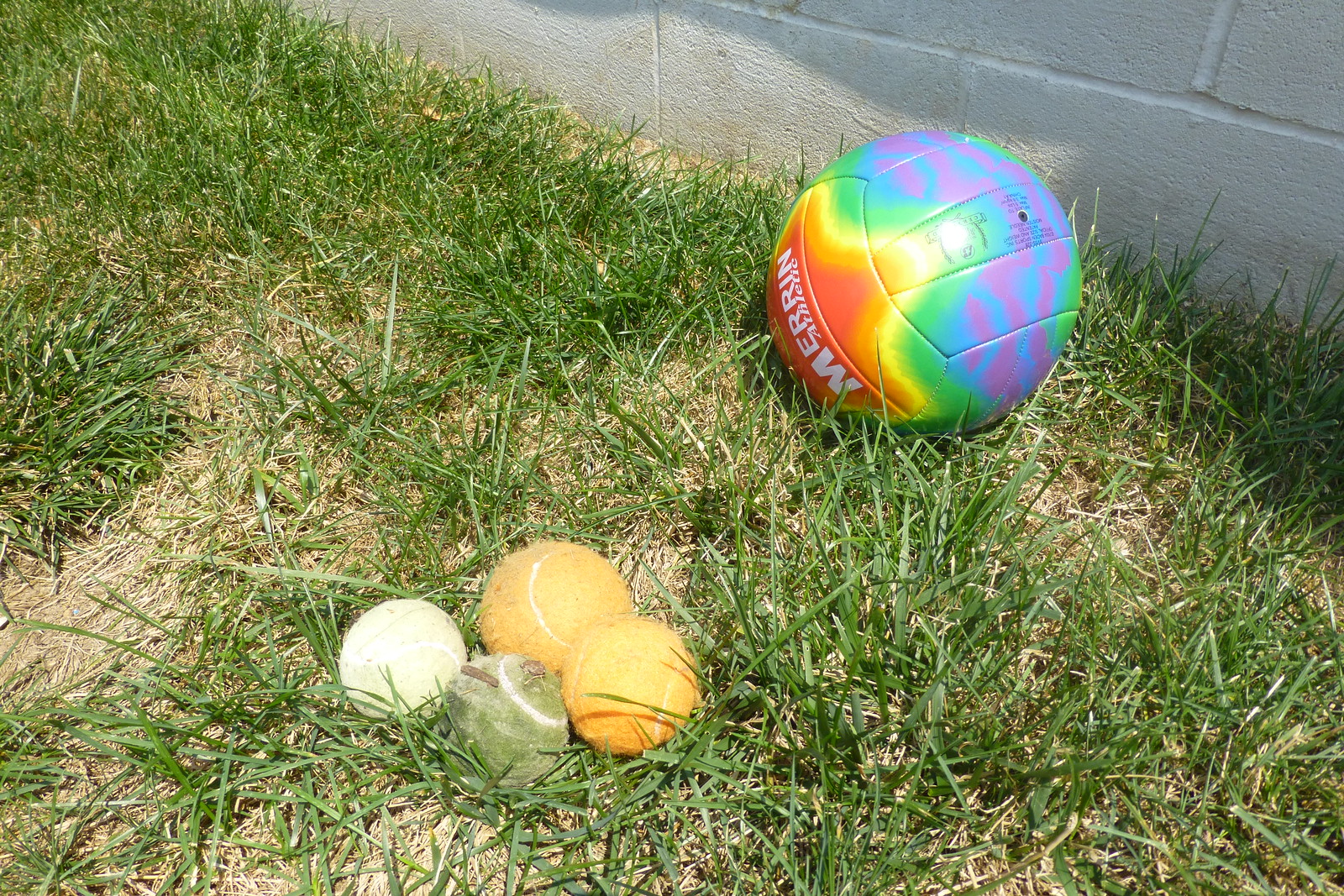In this photograph, five different balls rest on a patch of grass that appears dry and unhealthy, with significant brown areas. Four of the balls are tennis balls, each a different color: one green, one whitish, and two orange. These tennis balls are clustered together in the foreground near the center of the image. Slightly behind and to the right of the tennis balls is a vibrant, tie-dye rainbow-colored volleyball with the wording "Marin Athlete" on it, featuring a large red star. This ball stands out prominently against a white concrete cinder block wall, which serves as the backdrop in the upper right corner of the frame. The combination of these colorful balls and the contrasting background creates a visually interesting scene, evoking a playful and relaxed atmosphere.